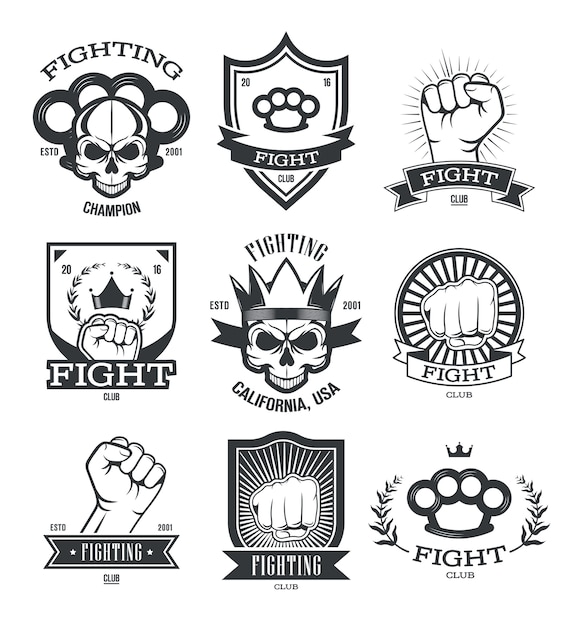This image features a series of nine black and white logos, each designed for a fight club, arranged in a three-by-three grid against a white background. The designs prominently feature recurring elements like fists, brass knuckles, skulls, crowns, and laurels, emphasizing the theme of fighting and combat. 

1. The first logo combines a skull with brass knuckles and includes the text "Fighting Champion Esto 2001."
2. The second logo showcases a shield with brass knuckles, a banner that reads "Fight Club," and the year "2016."
3. The third logo features a raised fist surrounded by striking marks and a ribbon stating "Fight Club."
4. The fourth logo, also shield-shaped, incorporates a crowned fist and laurels, with the text "2016 Fight Club."
5. The fifth logo portrays a skull wearing a crown, along with the words "Fighting California USA Esto 2001."
6. The sixth logo depicts a fist encircled by a radiant aura and a white banner reading "Fight."
7. The seventh logo shows a raised fist with a banner beneath it that says "Fighting Club 2001 Esto."
8. The eighth logo is a shield containing a central fist design and a banner stating "Fighting Club."
9. The ninth logo features brass knuckles topped by a small crown, flanked by laurels, and a banner reading "Fight Club."

All logos are rendered in black line work, giving them a stylized, hipster aesthetic suitable for a boxing gym or fight club.